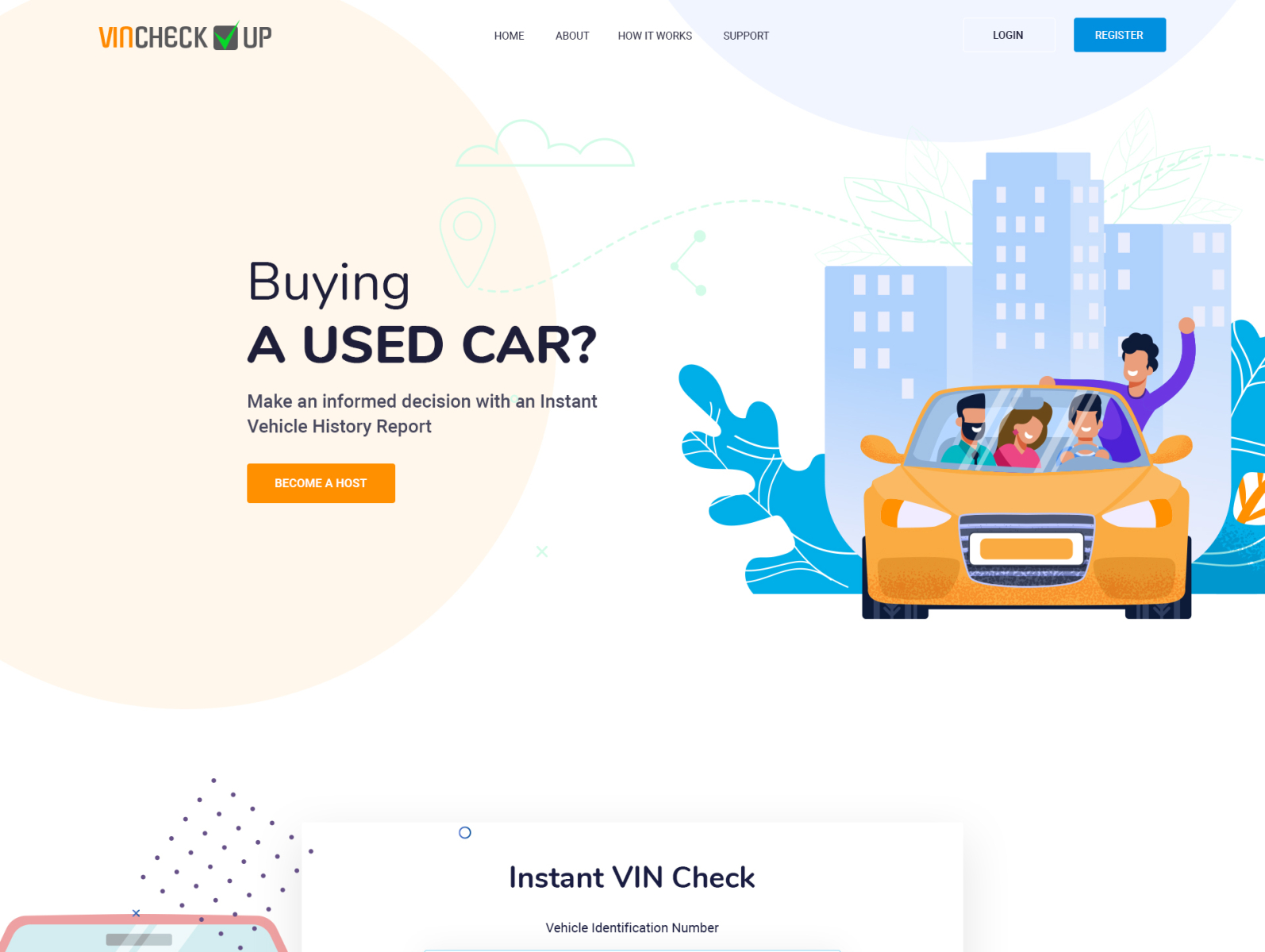At the top of the image, there is a header with the text "VIN Check" accompanied by a black square containing a green checkmark. To the right of this, there are navigation options labeled "Home," "About," "How it Works," "Support," and "Login." A blue button labeled "Register" is also present in this area. On the left side, there is a striking pink circle containing the tagline, "Buying a used car? Make an informed decision with an instant vehicle history report." Below this tagline, there's an orange button labeled "Become a Host."

On the right side of the image, an illustration features an urban skyline background with stylized blue elements that resemble splashing water. In the foreground, an orange car is prominently displayed with four passengers inside. One of the passengers, seated in the back seat on the driver's side and wearing a purple shirt, is leaning out of the window with their arm extended. Below this illustration, the text "Instant VIN Check," with a description labeling it as the "Vehicle Identification Number," is displayed. To the left of this text, there is a series of dots and a square.